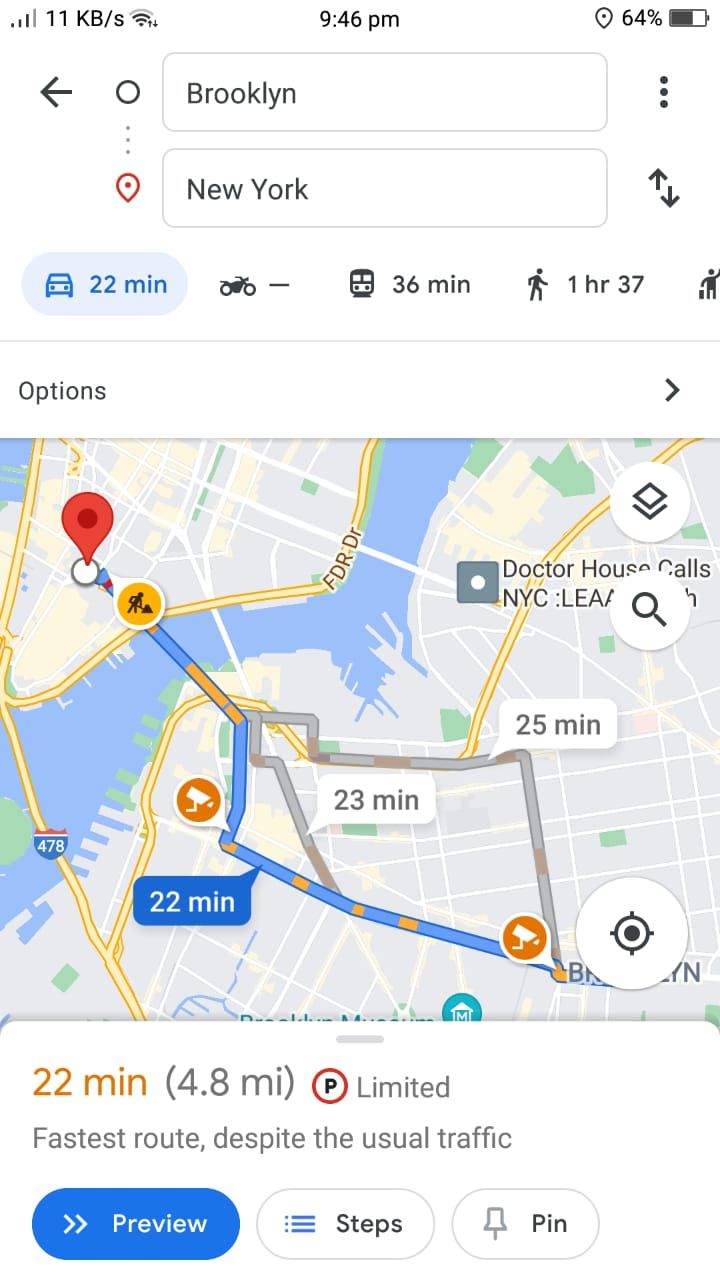Screenshot of Google Maps on a Smartphone at Night

This image captures a screenshot of Google Maps as viewed on a smartphone, evidenced by the status bar displaying 11 kilobytes per second data usage on the top left, the current time of 9:46 PM at the top center, and a 64% battery level at the top right. The user is looking up directions from Brooklyn to New York, and the map outlines various modes of transportation.

Prominently, the app indicates a 22-minute travel time by car for the 4.8-mile trip. Although no time is shown for motorcycles, the bus route is estimated to take 36 minutes, and walking would take approximately an hour and 37 minutes. There's a taxi icon visible as well, though details for this option and other modes aren't provided.

Below the transportation details, there's an options bar for further engagement, including a clickable blue "Preview" button, alongside "Steps" and "Pin" in white. The map itself highlights the route from Brooklyn to New York, displaying two orange camera icons and a note stating that parking is limited. The information confirms that the suggested route is the fastest, despite usual traffic conditions.